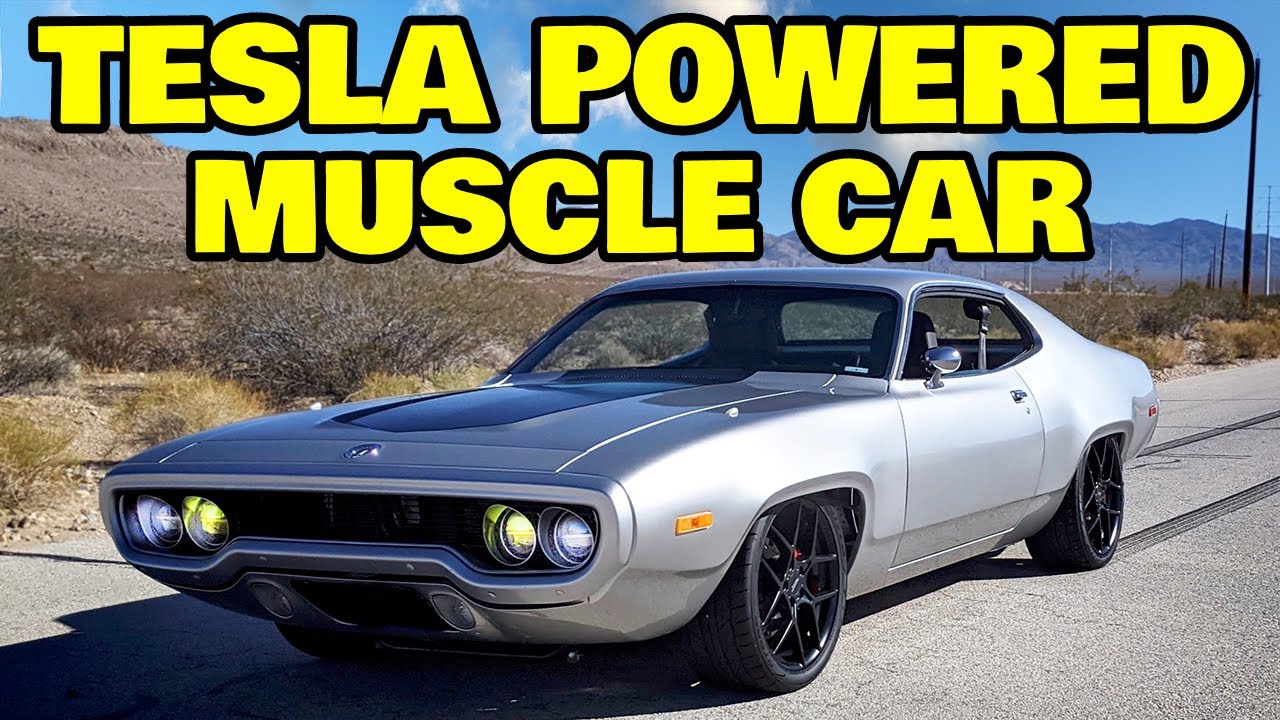A striking photograph showcases a sleek, gray muscle car prominently facing left on a weathered concrete road. **In bold neon yellow letters with a black border, the text "Tesla powered muscle car" dominates the top third of the image**. The car, boasting a sleek design with a long front and short back, features a black stripe down the middle of its hood. It has two doors and a black interior, while its headlights—two white and two yellow—shine brightly. The vehicle sits on black tires with black rims, and to its right, behind the car, black rubber marks stain the road. The backdrop includes a bright blue sky with white clouds, distant brown mountains, dried shrubs, and several power poles and lines stretching into the horizon.